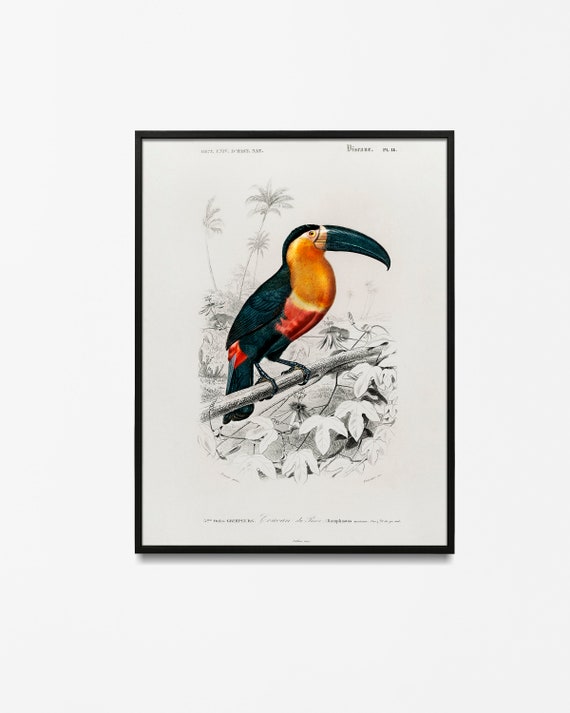The image is a detailed drawing set against a white background within a thin white mat and a black frame, hanging on a white wall. The central focus of the artwork is a vibrant parrot, perched on a branch, rendered in bright hues of orange, red, yellow, and green. The parrot's intricate colors starkly contrast with the grayscale surroundings. The bird, with a black beak and a mostly black tail, is perched on a branch amidst a backdrop featuring pencil-sketched elements, including branches, flowers, and several palm trees, evoking a tropical environment. There is small, hard-to-read text both at the top left and right, as well as at the bottom, with the latter in cursive, further contextualizing the scene. The overall composition juxtaposes the parrot's vivid plumage with the monochrome sketch, emphasizing its natural habitat.